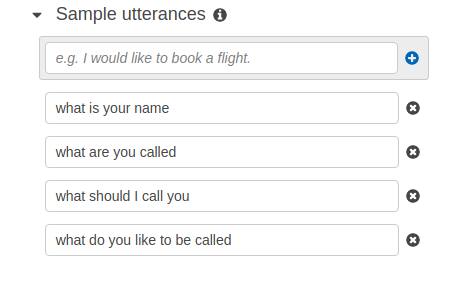This screenshot captures a section of a user interface, presumably from a web application with a white background. In the top left corner, there is a small, upside-down black triangle, about the size of a lowercase letter, next to a capital "S" that signifies the word "Sample". To its right, there is a black circle with a white lowercase "i" inside, indicating additional information. 

Below this header, there is a search bar outlined with a gray border, featuring placeholder text that reads "e.g., I would like to book a flight". Adjacent to the right side of the search bar, there's a light gray square containing a blue circle with a white plus icon in its center.

Underneath this, there is a series of search bars, each with different placeholder texts:
1. "What is your name" - accompanied by a black circle with a white "X" on the right side, outside of the search bar.
2. "What are you called" - again, paired with a black circle with a white "X" on the right, outside of the search bar.
3. "What should I call you" - similarly, with a black circle featuring a white "X" on the right side.
4. "What do you like to be called" - this final search bar also has a black circle with a white "X" on its right side.

All placeholder texts in the search bars are written in lowercase letters. The black circles housing white "X" icons consistently appear to the right of each search bar, serving as clear points for deleting or removing the entries.